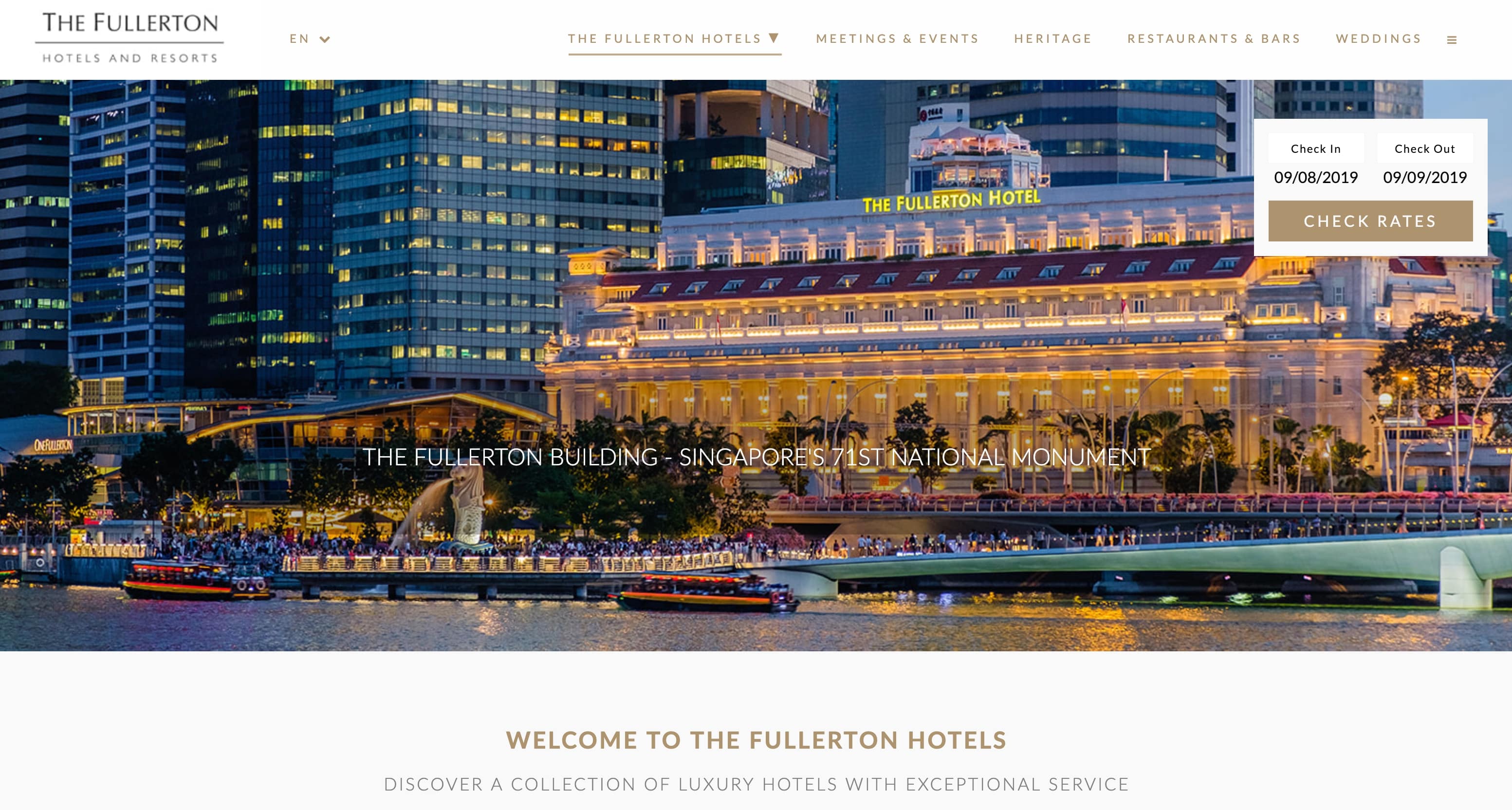This horizontal image, sourced from a website, provides a detailed view of The Fullerton Hotel's online presence, accessible via computer or smart device. The top portion of the image features a white navigation bar against the user's computer screen background. On the left side of the navigation bar, the text reads "THE FULLERTON" in bold, uppercase black letters with an underline, followed by "Hotels and Resorts." An option to select and change the language is available, with English currently selected.

The navigation bar offers various clickable options including "The Fullerton Hotels" (underlined), "Meetings and Events," "Heritage," "Restaurants and Bars," "Weddings," and a hamburger menu (three horizontal lines) for additional options.

Below the navigation bar is a scenic photograph showcasing a view across the river towards The Fullerton Hotel, with small boats visible on the water. Text overlaying the image declares "The Fullerton Building, Singapore's 71st National Monument."

In the upper right-hand corner of the image, a check-in/check-out booking box displays the dates "Check-in: 9-8-2019" and "Check-out: 9-9-2019" alongside a prominent brown button labeled "Check Rates" in white text.

Beneath the image, a light gray section warmly welcomes visitors with the message: "Welcome to The Fullerton Hotels." It further entices potential guests with the promise to "Discover a collection of luxury hotels with exceptional service." This comprehensive design effectively invites viewers to explore and experience the opulence of The Fullerton Hotel.